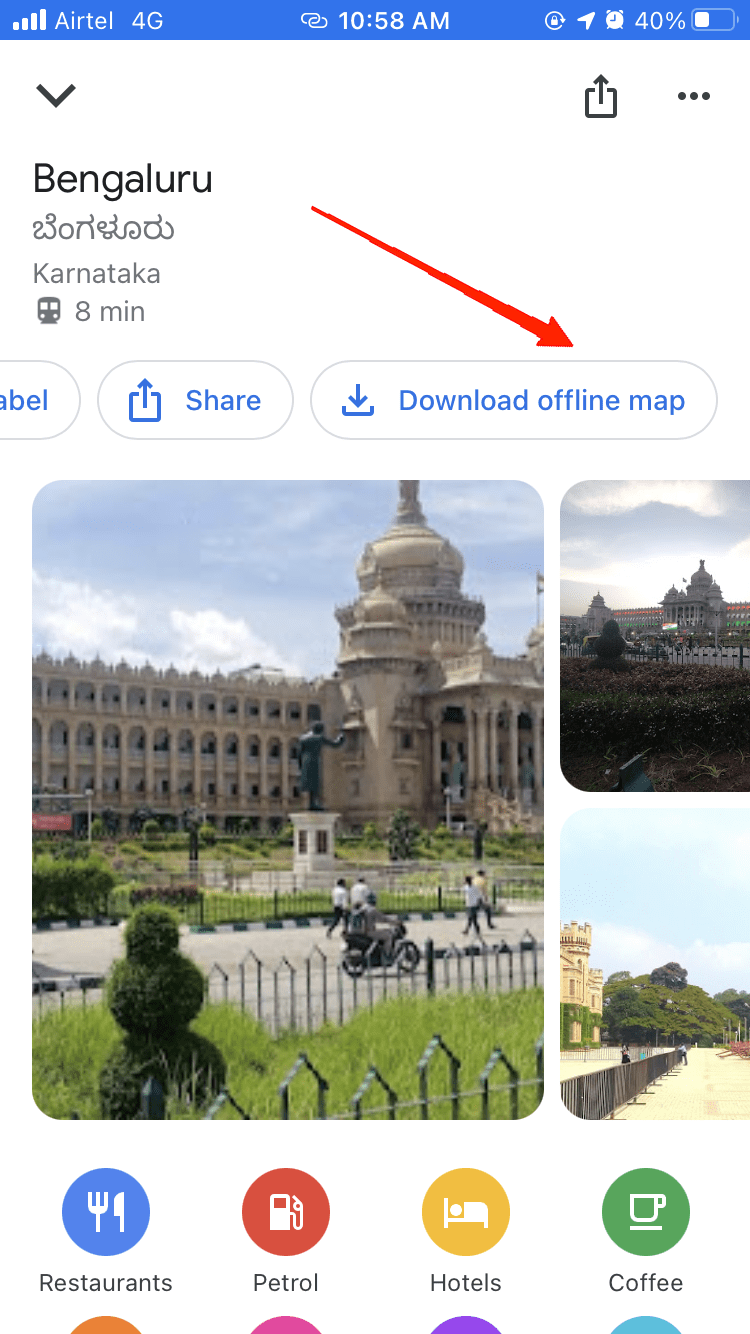Screenshot from a mobile phone displaying a map application. At the top, the blue status bar includes various icons and information: a full mobile signal, the network name 'Airtel 4G,' the current time '10:58 a.m.,' and icons indicating active location sharing, an alarm, and a battery level at 40%. Below the status bar, a white rectangle with 'Bangalore' written in black font appears, followed by text in a non-English script. Beneath this, there's a bus icon with '8 minutes' next to it. A red arrow points diagonally downward to a black oval with 'Download offline map' written in blue font inside it. At the bottom of the screen, three photos of the area are visible.